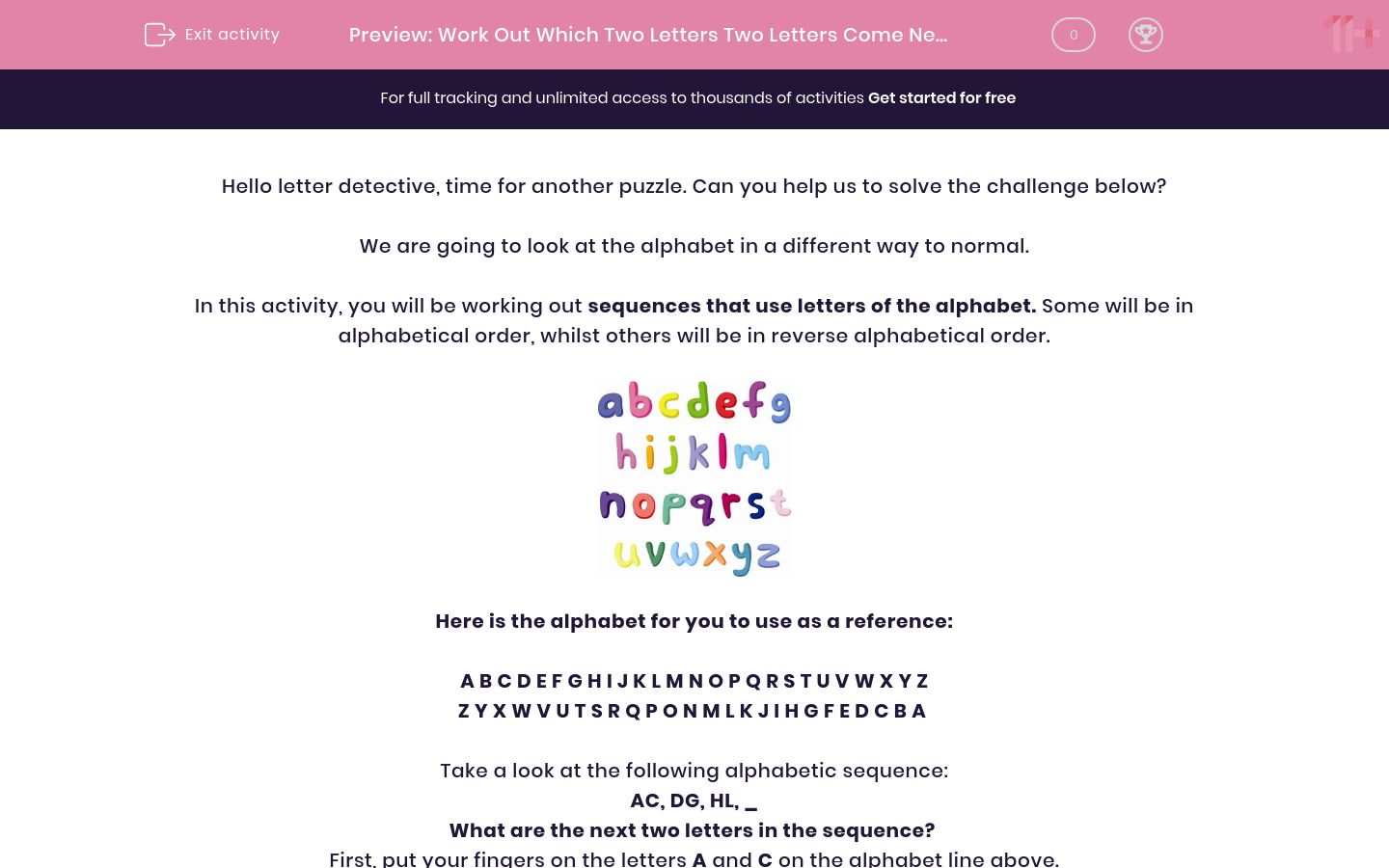This is a detailed screenshot from an educational website. At the very top, there is a navigation bar with a button on the left corner to exit the activity. It has a label that says "Preview," and the activity title reads: "Work out which two letters come ..." with an ellipsis indicating continuation. A button with the number '0' and a trophy icon is on the same bar, and in the upper right corner, it displays "11+" signifying the appropriate age group for the activity.

Below this bar, there is a prominent navy blue button with a call to action: "For full tracking and unlimited access to thousands of activities, get started for free," written in bold text. Beneath this, a friendly greeting says, "Hello Letter Detective, time for another puzzle. Can you help us to solve the challenge below? We are going to look at the alphabet in a different way to normal."

The instructions for the activity follow, introducing the user to puzzling out sequences using alphabet letters. It explains that some sequences will be in alphabetical order, while others will be in reverse.

An image of the full alphabet is provided for reference, captioned with: "Here's the alphabet for you to use as a reference." The activity continues with: "Take a look at the following alphabetic sequence: A, C, D, G, H, L, then a blank. What are the two letters of the sequence?" It also instructs the user to: "First put your fingers on the letters A and C on the alphabet line above."

The whole background of the website has a minimalistic design in white, contributing to the overall clean and focused appearance of the page.